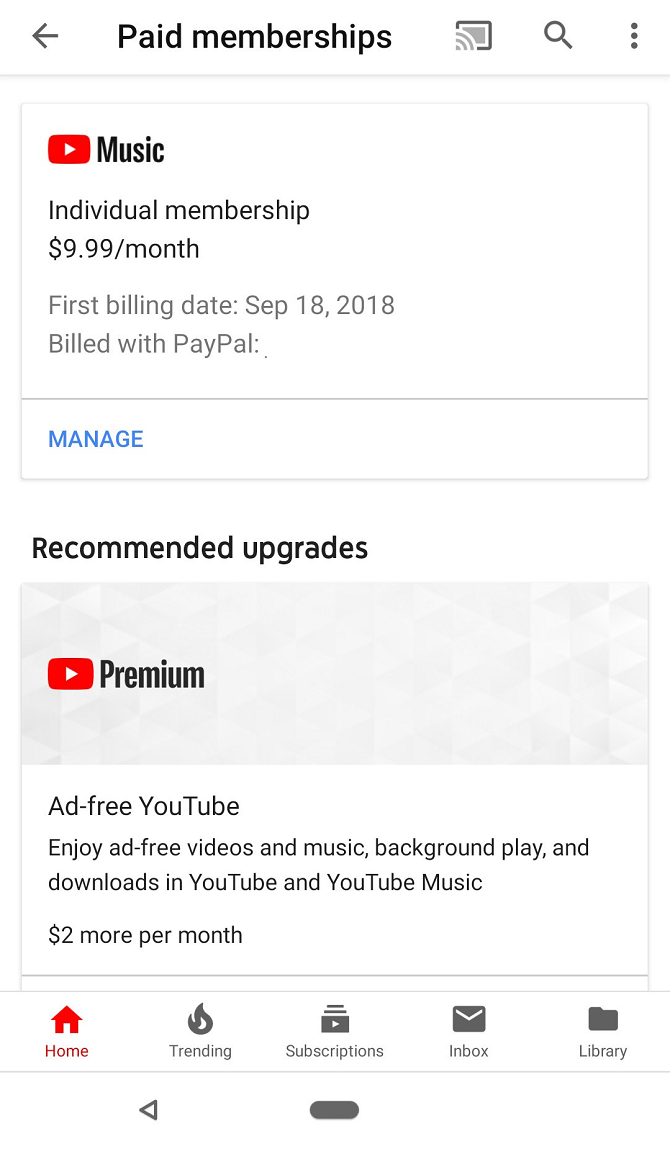**Detailed Caption:**

This image appears to be a screenshot taken from a mobile device, showing the user interface of the YouTube app under the "Paid Memberships" section. In the top-left corner of the screen, there is a back arrow, followed by the text "Paid Memberships". Adjacent to it, there is a screencast icon, a search icon, and three vertical dots indicating an expandable menu.

Below this, the screen is divided into sections. The first section features a rectangle on the left, showcasing the YouTube logo with the word "Music" beside it. This section provides details of an "Individual Membership" priced at $9.99 per month. The membership's first billing date is noted as September 18, 2018, and the payment method is listed as "Billed with PayPal". A horizontal line separates this section from the text below. There is a blue hyperlink labeled "Manage" for users to manage their subscriptions.

Beneath this, there is a section titled "Recommended Upgrades" which includes the YouTube Premium logo. This section highlights added benefits such as ad-free videos and music, background play, and downloads across YouTube and YouTube Music. It also mentions that these additional features are available for an extra $2 per month.

The bottom of the screen features a clickable toolbar with icons labeled "Home", "Trending", "Subscriptions", "Inbox", and "Library". The "Home" icon is highlighted in red, indicating it is currently selected, while the others are in gray. Below this toolbar, there's a thin clickable line on the left side featuring a back arrow to navigate backwards. The overall background of the screen is white, except for the YouTube Premium section which stands out.

This detailed layout captures the various elements and functionalities available on the YouTube app's "Paid Memberships" page, providing a comprehensive understanding of the user's options and navigation features.